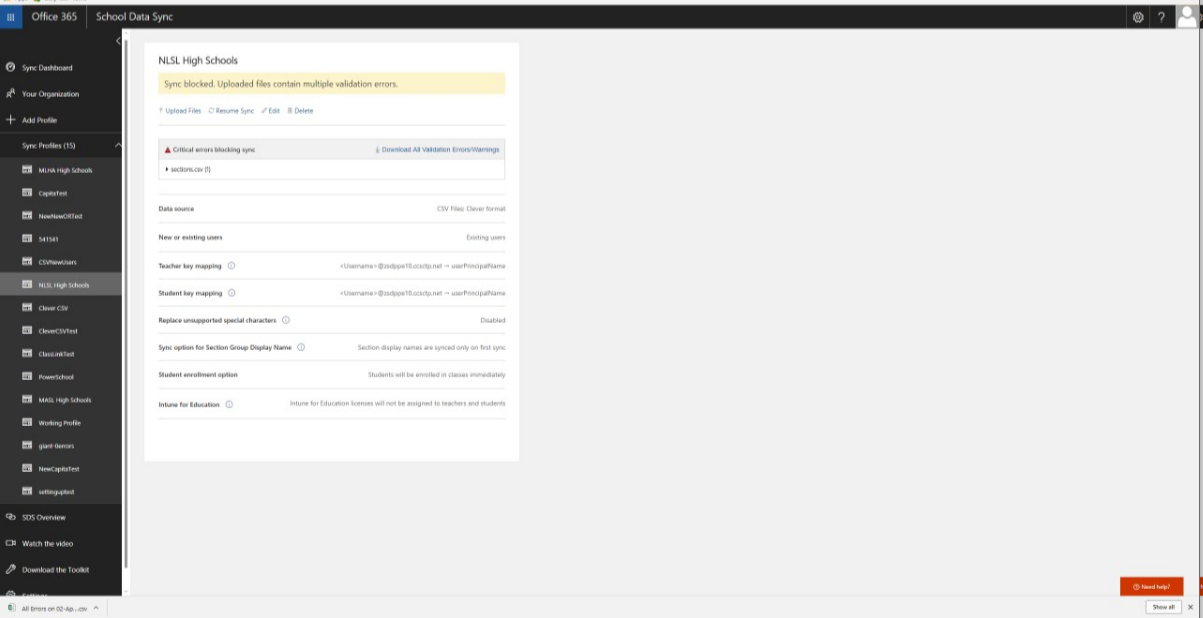The screenshot showcases the interface of Office 365's "School Data Sync" tool. In the top left corner, the title "Office 365, School Data Sync" is prominently displayed. Below this, on the uppermost menu bar, there are three icons: a settings gear, a question mark for help, and a generic profile icon symbolizing user settings.

A vertical black sidebar is situated on the left, containing a menu with white text. The visible menu options include "Sync Dashboard," "Your Organization," "Add Profile," and a few others that are not clearly readable due to their small size.

To the right of the black sidebar, a grey section features the text "NLSL High Schools" and highlights a significant status message: "Sync Blocked, Uploaded Files Contain Multiple Validation Errors." Accompanying this message, there is a red caution triangle icon emphasizing the critical nature of the issue.

Below the status message are several action buttons labeled "Upload Files," "Resume Sync," "Edit," and "Delete." Additional text in this area lists "Data Source," "New or Existing Names," "Teacher," and "Key Reporting," although some text remains illegible due to the small font size.

Towards the bottom of the interface, options such as "SOS Override" and "Watch the video" are listed, suggesting further support and instructional resources. The overall layout indicates areas for error management, file uploads, synchronization, and organization settings, though many finer details are challenging to discern from the provided screenshot.